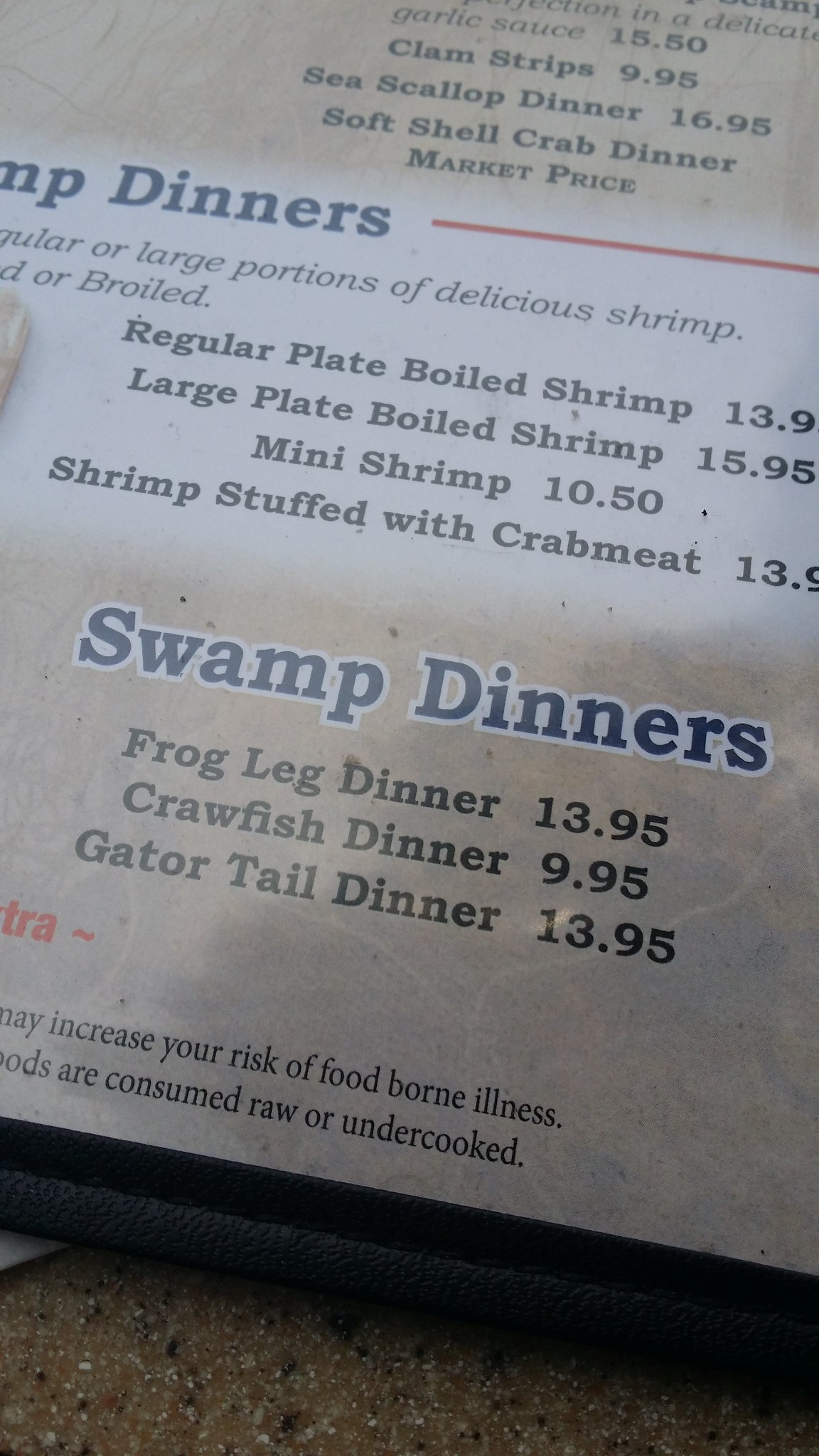This detailed indoor photograph captures a close-up of a menu printed on white paper. The visible portion of the menu presents about three or four lines of various seafood and exotic dishes, along with some remnants of text. At the top of the section, the menu lists "Clam Strips" for $9.95, "Sea Scallop Dinner" for $16.95, and "Soft Shell Crab Dinner" at market price. Following these entries, a larger font highlights a category titled "XXX Dinners" (the first word is obscured), separated by a horizontal red line. Below, the readable text boasts about "larger portions of delicious shrimp," going on to list boiled shrimp options such as "Regular Price Boiled Shrimp" for $13.90, "Large Platter Boiled Shrimp" for $15.95, "Mini Shrimp" for $10.50, and "Shrimp Stuffed with Crab Meat" for $13.90. 

Further down, another category titled "Swamp Dinners" appears in larger blue font. This section details "Frog Leg Dinner" for $13.95, "Crawfish Dinner" for $9.95, and "Gator Tail Dinner" for $13.95. At the very bottom, in finer print, a warning advises that consuming raw or undercooked food increases the risk of foodborne illness. The right side of the image fades into darkness while the lower left corner shows part of a table, providing a subtle hint of the restaurant’s ambiance.